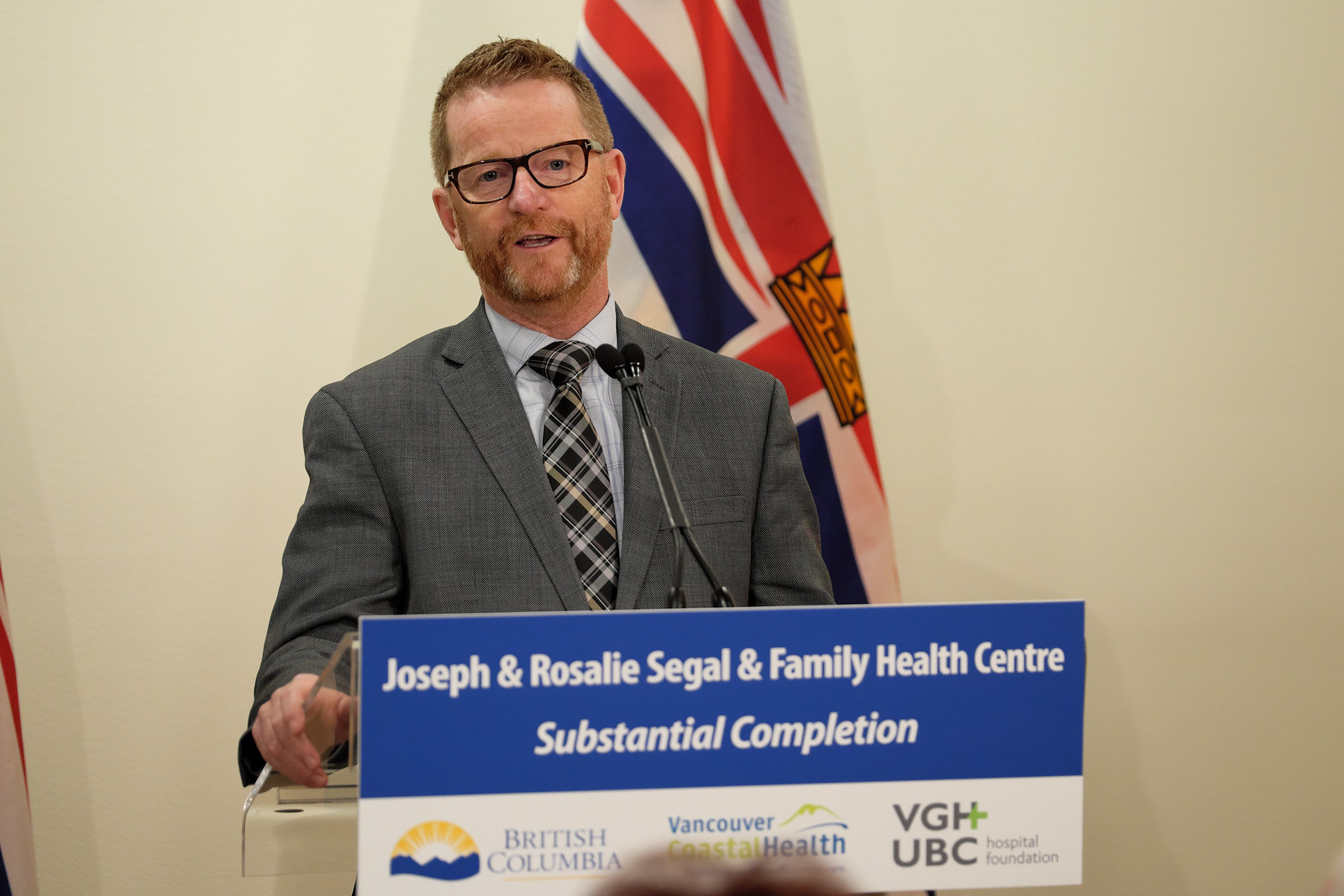The image features a man standing behind a podium, slightly left of center in the frame, delivering a speech into a small microphone. The man, who appears to be in his late 40s to mid-50s, has a short haircut with reddish brown hair, a mustache, a slight beard with some gray, and is wearing dark-rimmed glasses. He is dressed in a dark-colored suit jacket, a light-colored shirt, and a blue plaid tie. The podium in front of him has a sign that reads "Joseph and Rosalie Siegel and Family Health Center" with "Substantial Completion" printed beneath it. The sign also includes logos and text related to British Columbia, Vancouver Coastal Health, and VGH-UBC, presented on a blue and white background. Behind him, to his left, a flag with red, white, and blue colors, featuring an orange insignia in the middle, is displayed against a white wall. Additionally, part of a person's head is visible in the foreground, centered at the bottom of the sign.